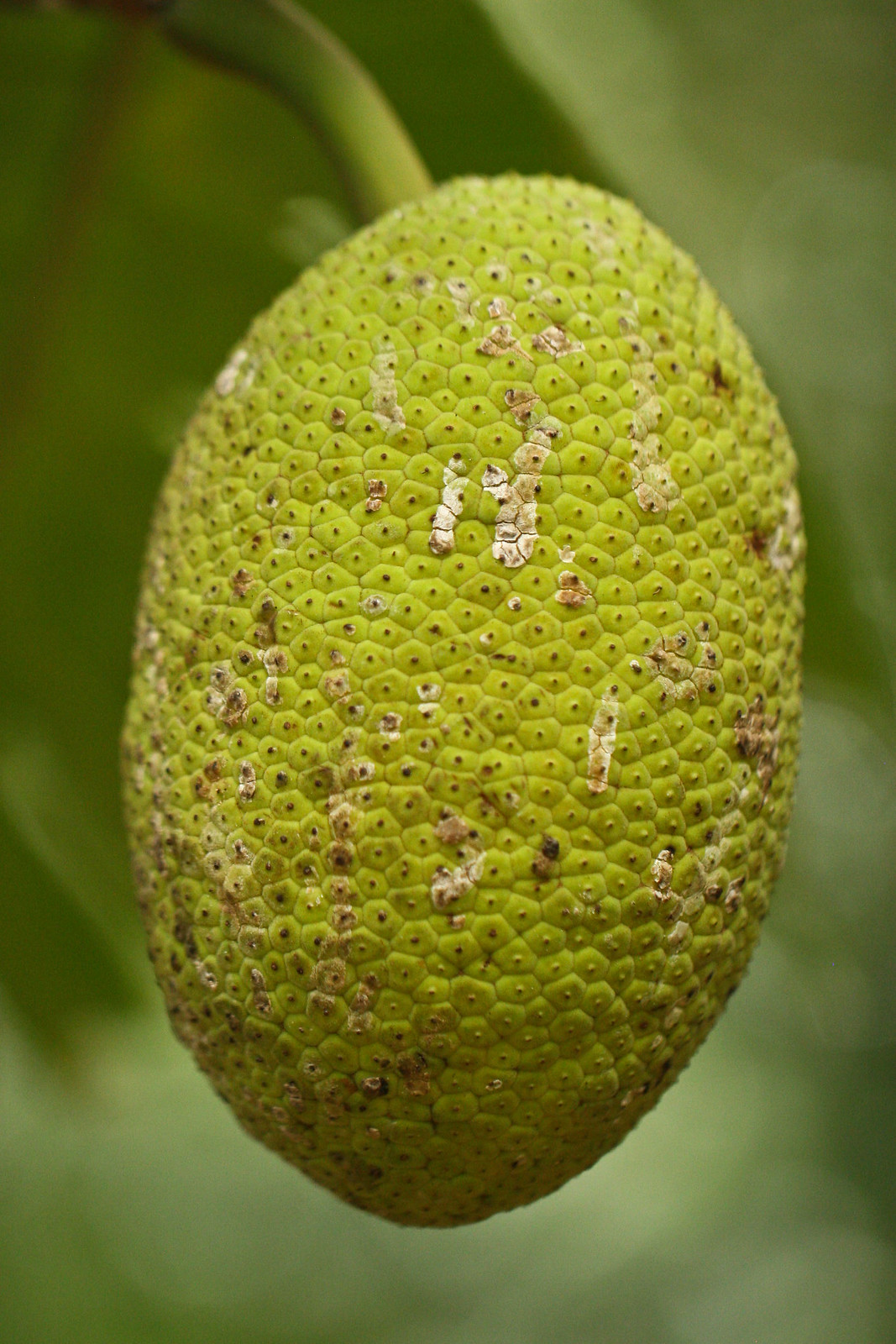This full-color photograph, taken outdoors in the daytime, features a detailed close-up of an egg-shaped, green fruit attached to a long stem emerging from the upper left corner of the image. The fruit, about the size of a large egg, has a patterned surface with small squares of green and brown dots, along with various white, random spots that could be indicative of mildew, mold, or bird droppings. There are also small, white, worm-like structures scattered across the fruit, possibly the beginnings of blossoms. The background is artistically blurred, showcasing out-of-focus green leaves and trees, enhancing the focus on the central fruit. The image, rectangular in shape, exudes an artistic quality, highlighting the natural, textured details of the mysterious fruit, which is likely not native to America.